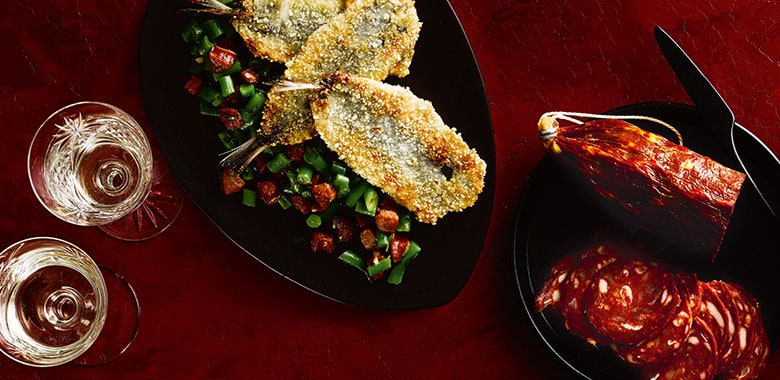This image captures a sophisticated appetizer spread set on a red polished table with visible cracks. At the center of the scene, two distinct plates rest side by side. On the left, a black oval plate features three crispy fried cutlets, possibly fish, arranged one atop another. Garnishing the plate are tiny, chopped green beans and perhaps cranberries, adding a burst of color. Nearby, two elegant aperitif glasses, either filled with a clear liquid or left empty, suggest a touch of class. To the right, a round black plate showcases a whole dry-cured summer sausage, partially sliced. The slices reveal a marbled texture typical of quality salami. A small serving spatula lies ready for use next to the unsliced portion. Collectively, the presentation, with its careful arrangement of various appetizers, portrays a refined pre-meal setup.